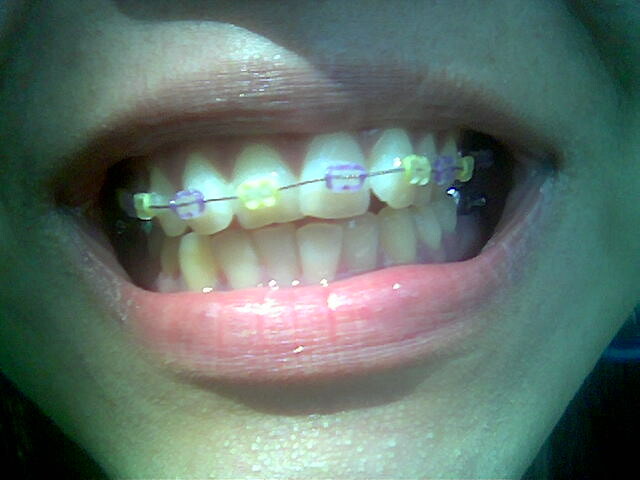This is a highly detailed, close-up photograph capturing the lower half of a Caucasian person's face, focusing on their mouth and teeth. The image spans from just below their nose, omitting their nostrils, down to just above the bottom edge of their chin. The person is holding their mouth open, revealing both the top and bottom rows of their teeth. The bottom teeth are clear and straight, with visible metal molars at the back. The top teeth are adorned with braces, which feature alternating yellow and purple squares attached to the teeth with a wire running through them. The person’s lips are pink and appear somewhat dried at the edges where they meet. There’s a noticeable glare on the teeth, suggesting a strong light source, while other areas are in shadow. Subtle details such as little bumps on the chin and the crease between the person's lips and cheek are also visible. The overall composition leaves little room for background, concentrating entirely on the intricacies of the mouth and braces.